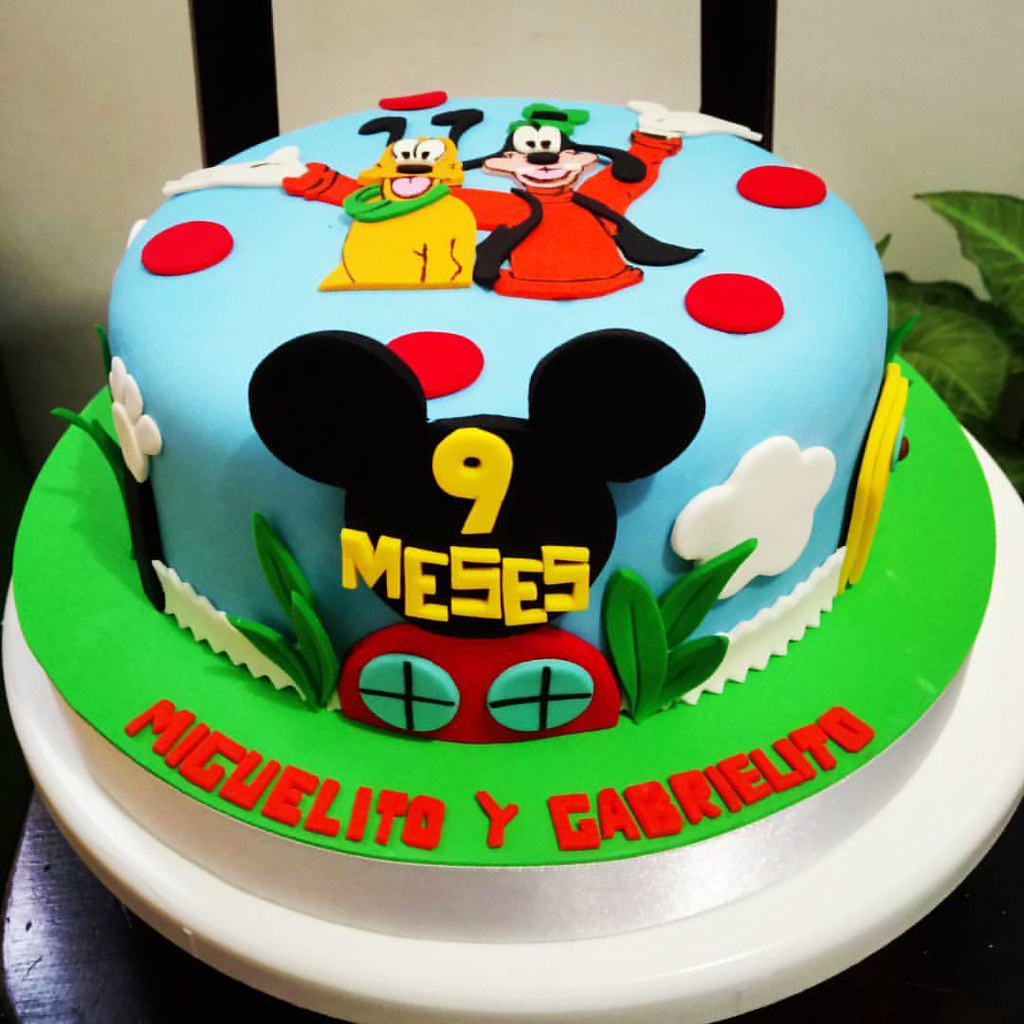This image showcases a meticulously decorated children's birthday cake, seemingly for twins Miguelito and Gabrielito. The cake resides on a white pedestal, which is placed atop a dark wood table. The cake itself is round, with a vibrant green fondant layer at the base that features the names "Miguelito y Gabrielito" written in bold red letters. Above, the cake is enveloped in a sky-blue fondant, adorned with fluffy white clouds and large red polka dots scattered across the surface.

Central to the design is a black silhouette of Mickey Mouse's head on the front, with the words "9 MESES" (9 months) written in yellow fondant, likely celebrating the twins' nine-month milestone. Mickey Mouse's iconic red shorts with two large buttons are also depicted.

The top of the cake is a lively scene: Goofy, donned in his characteristic green hat and red shirt, stands with arms joyously outstretched. Beside him is Pluto, the tan dog with big black ears and a green collar, exuding happiness with his tongue hanging out. The scene is completed with additional decorative elements, including fondant leaves, a white picket fence, and the green grass-like fondant base, bringing a whimsical, Disney-inspired environment to life. The background details include a house plant placed to the right of the cake, and the setting appears to be indoors, possibly against a beige wall.